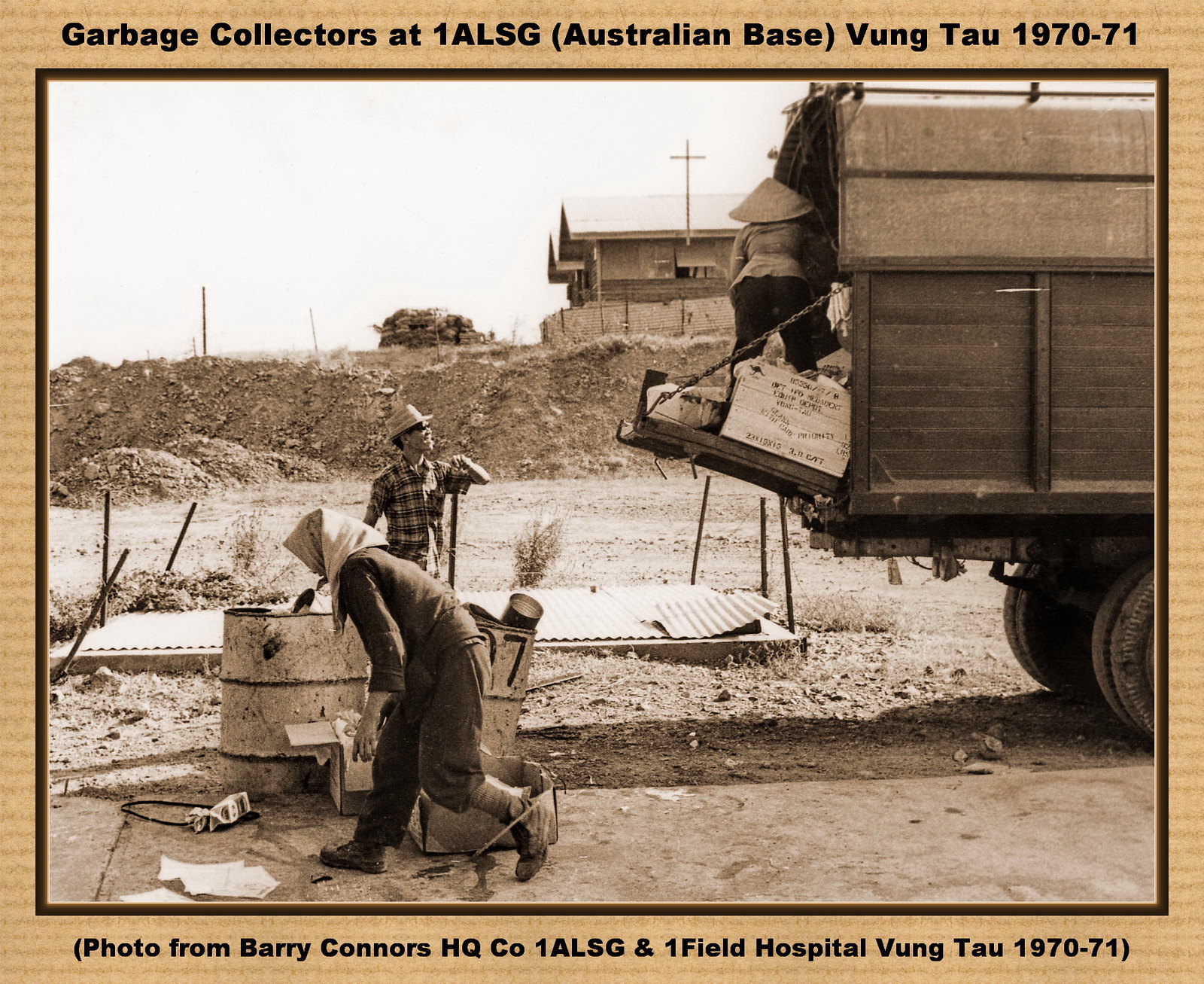**Garbage Collectors at 1ALSG, Australian Base, Vung Tau, 1970-71**

In this black and white photo, likely taken in Vietnam, two men are positioned towards the left side of the image. The man in the back is distinguished by his tall straw hat and checkered shirt as he looks towards the right. In front of him, a man wearing a white headscarf or babushka stands hunched over, facing left. Between them lie two large metal buckets, likely used for handling garbage.

On the right side of the image, a military garbage truck with its back door opened is visible. Standing inside the truck is a woman wearing a wide-brimmed triangular hat, appearing to sort or handle the boxes seen in the truck. The surrounding area consists mainly of dirt, with a noticeable dirt hill and building topped with sandbags in the background, suggesting a military installation setting.

The photo is bordered by a black frame, encased in an outer lighter brown border. Text above and below the picture reads: "Garbage Collectors at 1ALSG, Australian Base, Vung Tau, 1970-71" and "(Photo from Barry Connors, HQ, CO, 1ALSG and 1 Field Hospital, Vung Tau, 1970-71)."